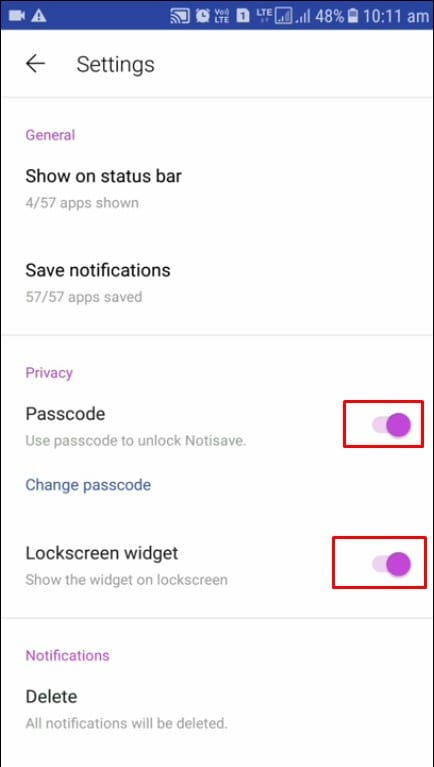The screenshot depicts a settings page from a smartphone, with a blue header and various interface elements. 

At the top, the status bar displays:
- A white camera icon on the left.
- A white triangle with an exclamation point.
- A line plot.
- 'LTE' in white text.
- A white rectangle with the number '1' inside it.
- Another 'LTE' symbol.
- Fully lit white service bars.
- A battery icon indicating 48% charge.
- The current time, '10:11 a.m.'

Below the status bar, the page background is predominantly white with a series of sections and options listed. 

**Details:**

- **Left Arrow:** There is a left-pointing arrow and the word "Setters" in black font.
- **Dividers:** A gray horizontal line runs across the interface separating different sections.
  
  **Sections:**
  
1. **General (in purple):**
    - Show Status Bar (in black)
    - 57/57 App Show (in gray)
    - Save Notifications (in black)
    - 57/57 App Saved (in gray)
  
2. Another gray horizontal line follows.
  
3. **Privacy (in purple):**
    - Passcode (in black)
    - Use passcode to unlock notice save (in gray)
    - Change Passcode (in blue)
    - Lock Screen Widget (in black)
    - Show the widget on the screen (in gray)
  
4. Another gray horizontal line follows.
  
5. **Notifications (in purple):**
    - Delete (in black)
    - All notifications will be deleted (in gray)

This detailed description captures the layout and content of the settings page on the smartphone, giving a clear depiction of the interface elements and their arrangement.